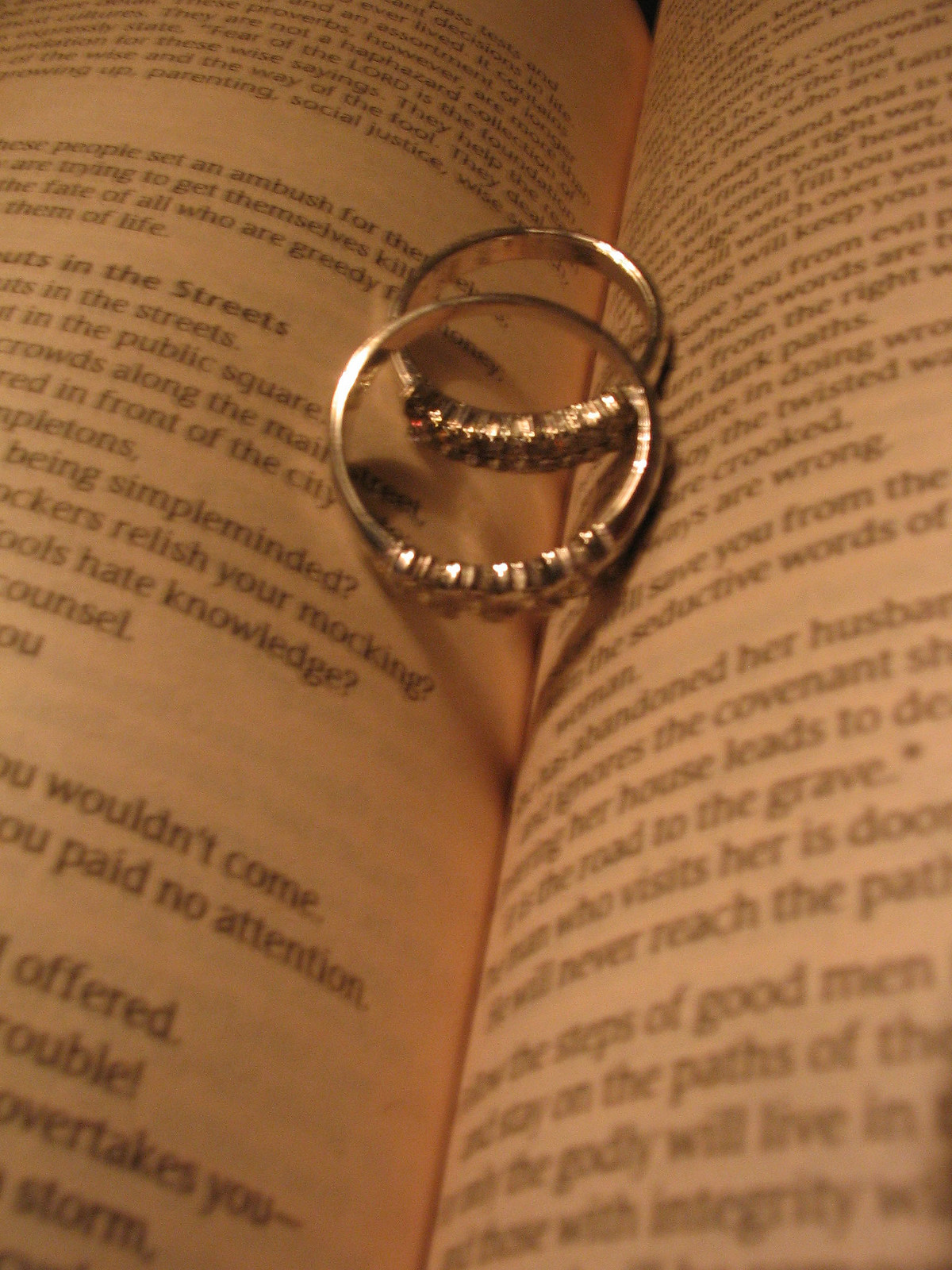The photograph features an open book with its yellowed pages spread out on a table, hinting at an indoor setting. In the crease where the two pages meet, there's a pair of shiny rings, overlapping in the center of the book. The rings, likely silver but possibly gold, are adorned with various gemstones, including clear and red stones, arranged in intricate rows. The text on the pages is partially visible and includes phrases like "in the streets," "public square," and other fragmented sentences, though the details are blurry and unclear. The main focus of the image is the intricate and sparkling rings positioned prominently in the middle of the book.